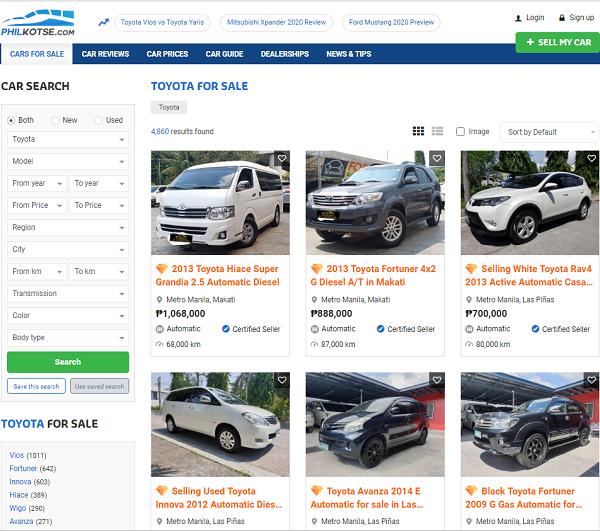### Detailed Caption:

The image showcases a dynamic car dealership website, prominently featuring the URL **philcottsey.com**. The header highlights several key sections: "Toyota Vicks vs. Toyota Yaris," "Mitsubishi Xpander 2020 Review," and "Ford Mustang 2020 Preview." Additionally, options for "Log In," "Sign Up," and "Sell My Car" are visible, encouraging user interaction. Notably, a green button stands out for certain actions.

Below the header, a blue navigation bar spans the width of the page, listing categories like "Cars for Sale," "Car Reviews," "Car Prices," "Car Guide," "Dealerships," and "News and Tips." This provides users with comprehensive information and options.

A car search tool is prominently placed, allowing users to filter by model, year, region, city, color, transmission, body type, and then execute their search by clicking a green search bar at the bottom. The results specifically list Toyotas for sale, including the count of available models such as Vicks and Frontrunners in parentheses.

Displayed beneath the Toyota listings are six diverse car images, each accompanied by descriptions in orange text. Details include the cars' locations, prices, and mileage. The showcased vehicles consist of a white van, a black SUV, a white SUV, another white SUV of the same model, a newer black SUV, and an additional black SUV, reflecting a variety of choices for potential buyers.